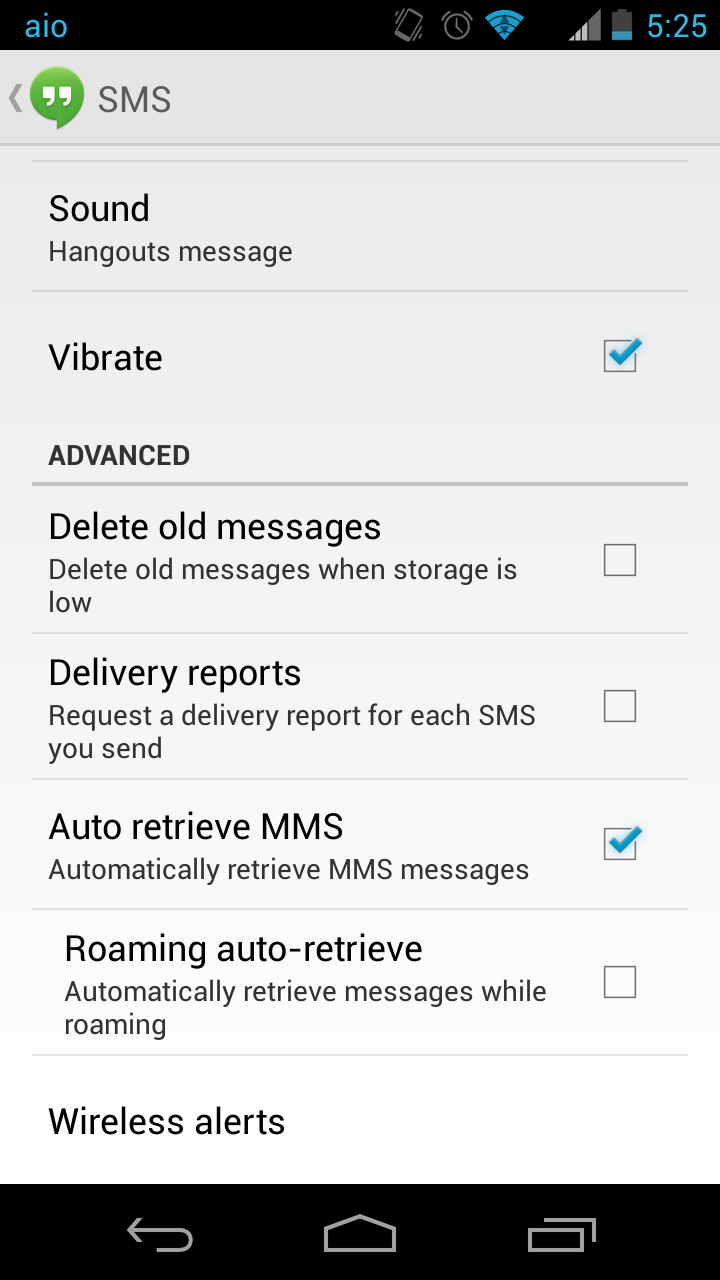The image showcases a screenshot of a settings interface, likely from a tablet or smartphone. The design features a light gray background with black text and various checkbox options. At the top of the screen, there's a black bar displaying "AIO" in blue, alongside system indicators such as the time (5:25), battery status, and wireless connection symbols.

Beneath this top bar, the main settings page begins with an "SMS" heading accompanied by a green icon. Following this are several notification options including "Sound" and "Hangouts message". Each of these options has a corresponding checkbox. For example, "Vibrate" has a checked box.

A section labeled "Advanced" includes various options:
- "Delete Old Messages": Delete old messages when storage is low (unchecked box).
- "Delivery Reports": Request a delivery report for each SMS sent (unchecked box).
- "Auto-Retrieve MMS": Automatically retrieve MMS messages (checked box in blue).
- "Roaming Auto-Retrieve": Automatically retrieve messages while roaming (unchecked box).

The last visible section in the screenshot is titled "Wireless Alerts".

Each setting is organized neatly, providing a clear overview of the user's messaging and alert configurations.